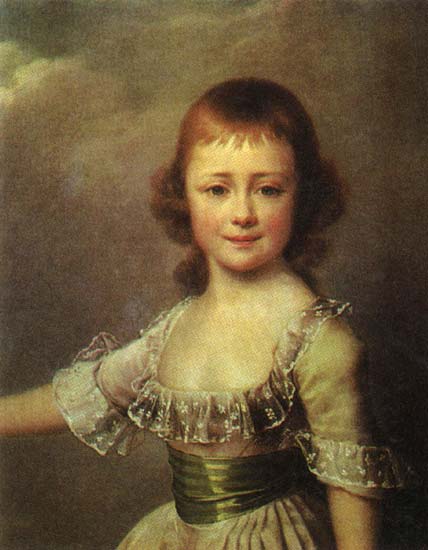The painting depicts a young girl with auburn, short hair neatly cut at the bangs, covering her ears, and curling slightly at the back near her neckline. She stands against a dark, somewhat somber backdrop that transitions from a darker hue at the bottom to a cloudy, twilight sky above, evoking a mysterious and timeless atmosphere. The girl, dressed in a period-style outfit reminiscent of the Renaissance or 18th to 19th-century fashion, wears a dress with a low neckline adorned with transparent frills extending to her elbows. A distinct bronze or golden sash cinches her waist, emphasizing the flared design of her dress, which extends out below the belt but is cropped at her upper thighs by the frame.

Her youthful face is finely detailed, showcasing a prominent nose and mouth, and she gazes directly at the viewer with a puzzled, somewhat perplexed expression. Despite her direct gaze, the girl is not smiling, encapsulating a mood that isn’t easily defined as happy or sad. The image has a warm yet muted, earthy palette accented with touches of green and red, delivering an overall photorealistic impression that enhances the painting's rich textures and lifelike quality.